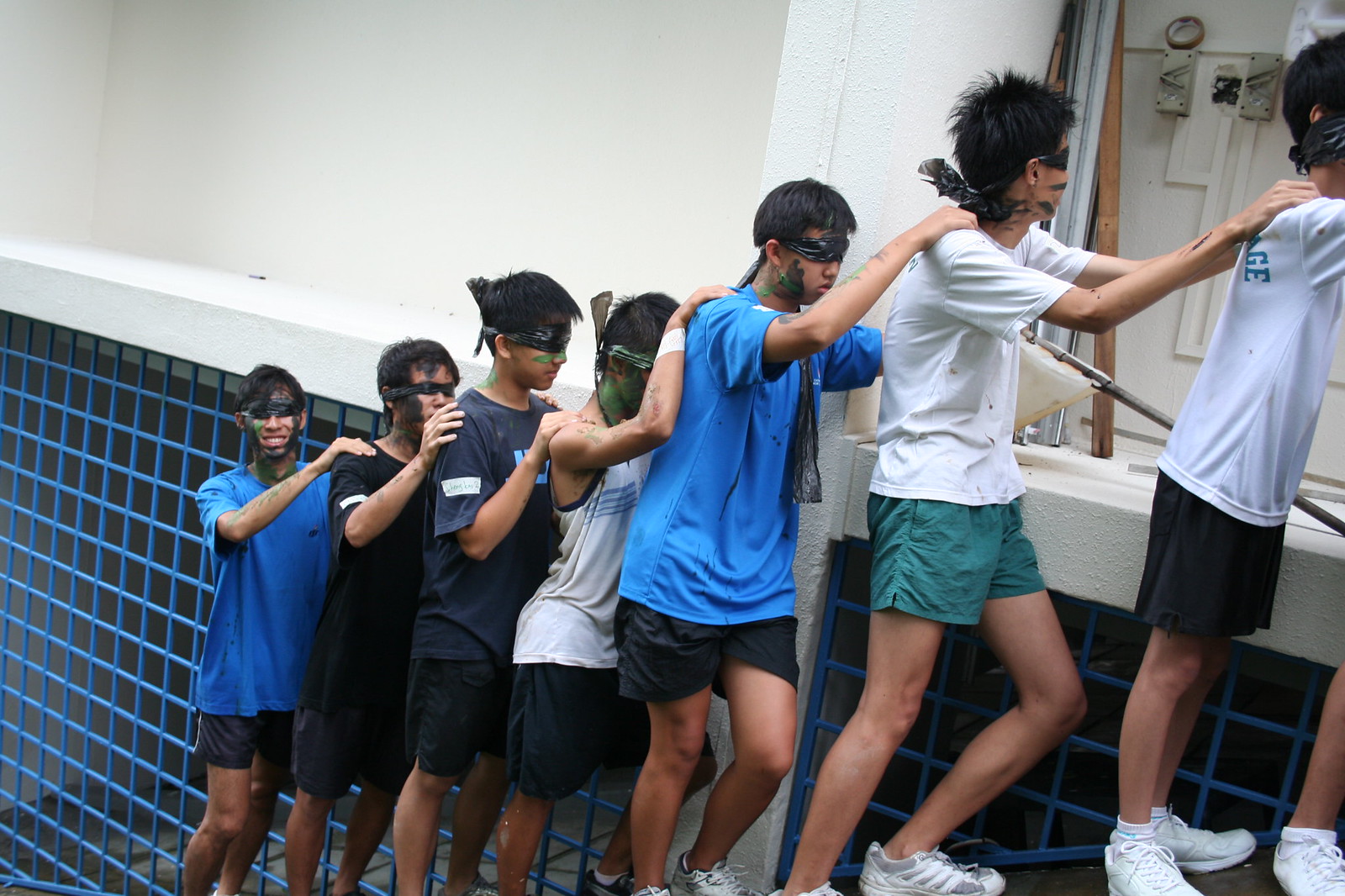In this detailed image, a group of seven teenage boys, aged around 15 to 17, are meticulously lined up in single-file formation with each boy placing his hands on the shoulders of the boy directly in front of him. They are all blindfolded, suggesting this could be a trust exercise or an advanced course involving obstacles. The boys are dressed casually in t-shirts, shorts, and tennis shoes, with subtle variations in their attire including blue, black, and white shirts, and green and black shorts.

The setting reveals the group as they navigate upwards, possibly towards a stage or further steps. They are positioned against a wall characterized by dark blue tiles with light blue crisscross lines forming squares, transitioning to a white column and an indented white wall further ahead. On the right, they appear to be heading towards an upper level. Behind the first boy in the line, there's a partially visible white wall adorned with potential fixtures like a clock or thermostat and a wooden object against it. This intricate description captures the boys' coordinated movement and the visually striking elements of their environment.